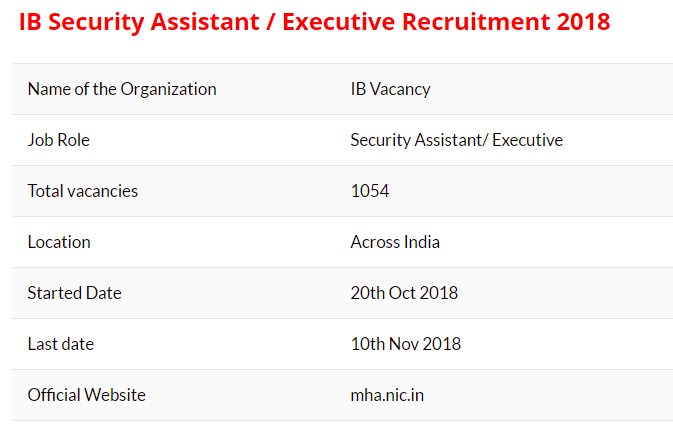The image is a slide from a PowerPoint presentation detailing the IBE Security Assistant and Executive Recruitment for 2018. The slide, with a white background and black and red text, prominently features the title "IB Security Assistant/Executive Recruitment 2018" in red Arial font at the top. This title is followed by a structured table that is organized into two columns and seven rows. Each row alternates between light gray and white shading, starting with the light gray at the top. 

The left column of the table lists the subjects: "Name of organization," "Job role," "Total vacancies," "Location," "Start date," "Last date," and "Official website." Corresponding information in the right column includes: "IBE Vacancy" for the organization name, "Security Assistant/Executive" for the job role, "1,054" total vacancies, "Across India" as the location, "20th October 2018" as the start date, "10th November 2018" as the last date, and "mha.nic.in" as the official website.

The slide provides a clear, organized overview of the recruitment details, ensuring that all critical information is easily accessible at a glance.